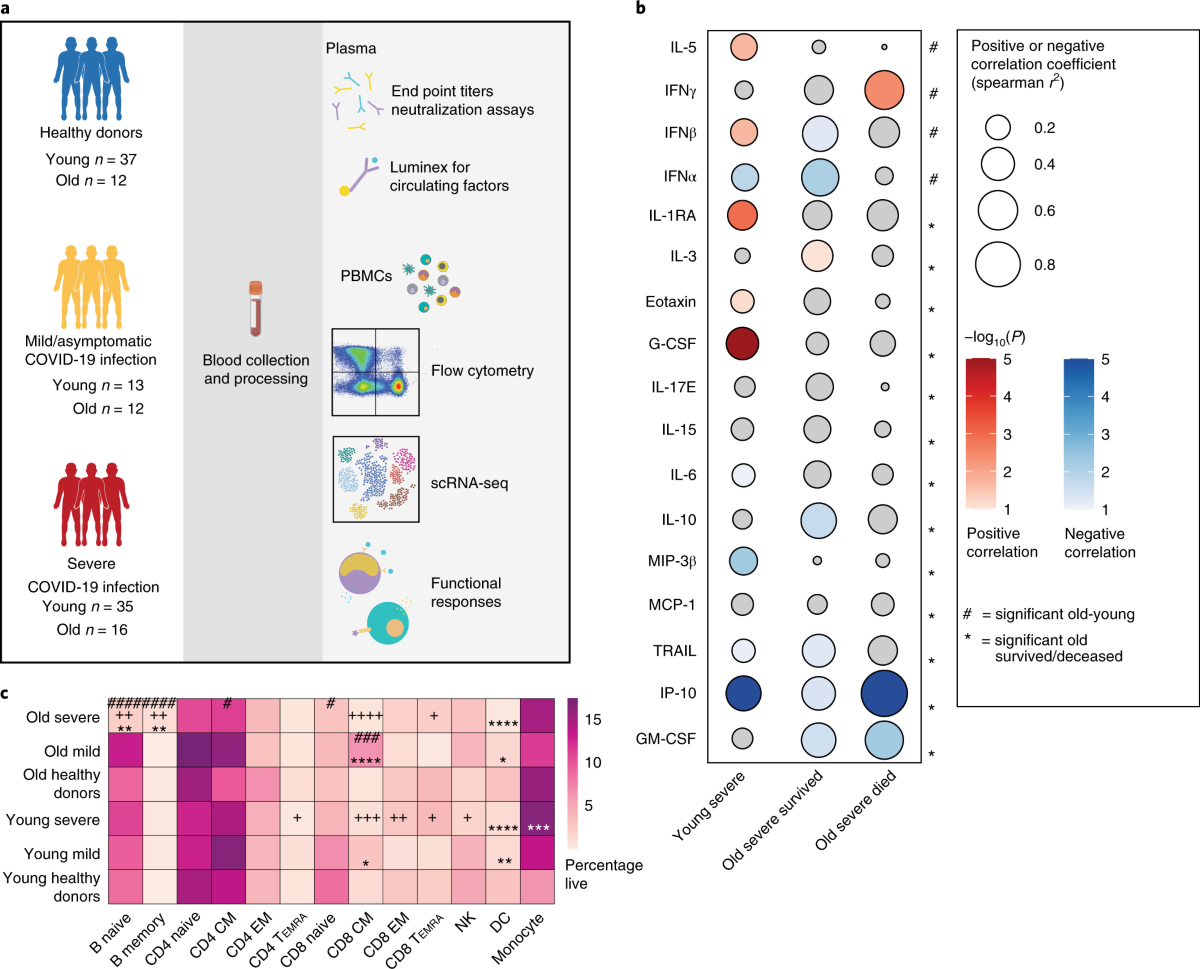The image appears to be a detailed infographic from a textbook that provides statistical and process information about COVID-19 infections. In the top left corner, three groups of people are depicted using colored silhouettes. The blue silhouettes represent 'Healthy Donors' with the subcategories 'Young (N=37)' and 'Old (N=12)'. Below that, yellow silhouettes indicate 'Mild/Asymptomatic COVID-19 Infection’, divided into 'Young (N=13)' and 'Old (N=12)'. The bottom row features red silhouettes for 'Severe COVID-19 Infection', categorized as 'Young (N=35)' and 'Old (N=16)'. An illustration beside these groups details the process of 'Blood Collection and Processing', leading to 'Plasma', illustrating various analytical techniques like 'flow cytometry' and 'neutralization assays'. Additional charts in the image display various data points, including a chart with purple and pink squares and another with colored dots indicating outcomes for 'Young Severe', 'Old Severe Survived', and 'Old Severe Died'. The final chart mentions the 'positive or negative correlation coefficient (Spearman)’. This structured layout conveys an extensive overview of different infection severities and associated analytical methods for blood plasma processing.